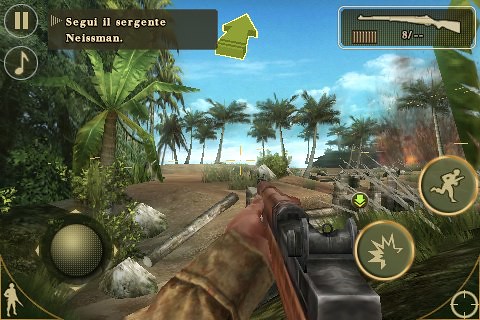The image is a screenshot from a first-person military-style shooter video game set in a tropical location. The player character is visible from a first-person perspective, holding a rifle with a brown and black metal frame. The character's left arm, clad in a dirty whitish-yellow sleeve resembling a military uniform, extends into view. The scene depicts a dirt path bordered by palm trees and dense foliage, suggesting a beach or tropical environment under a blue sky with thin white clouds. On the right side of the image, there is a distant fire or explosion. The game's HUD (Heads-Up Display) includes a green directional arrow at the top center, urging the player to follow a path and accompanying text in Italian, "Segui il Sergente Neisman." The top right corner shows an ammo count, while icons around the edges include a circular button on the left, and two buttons on the right depicting a running man and an explosion, respectively.